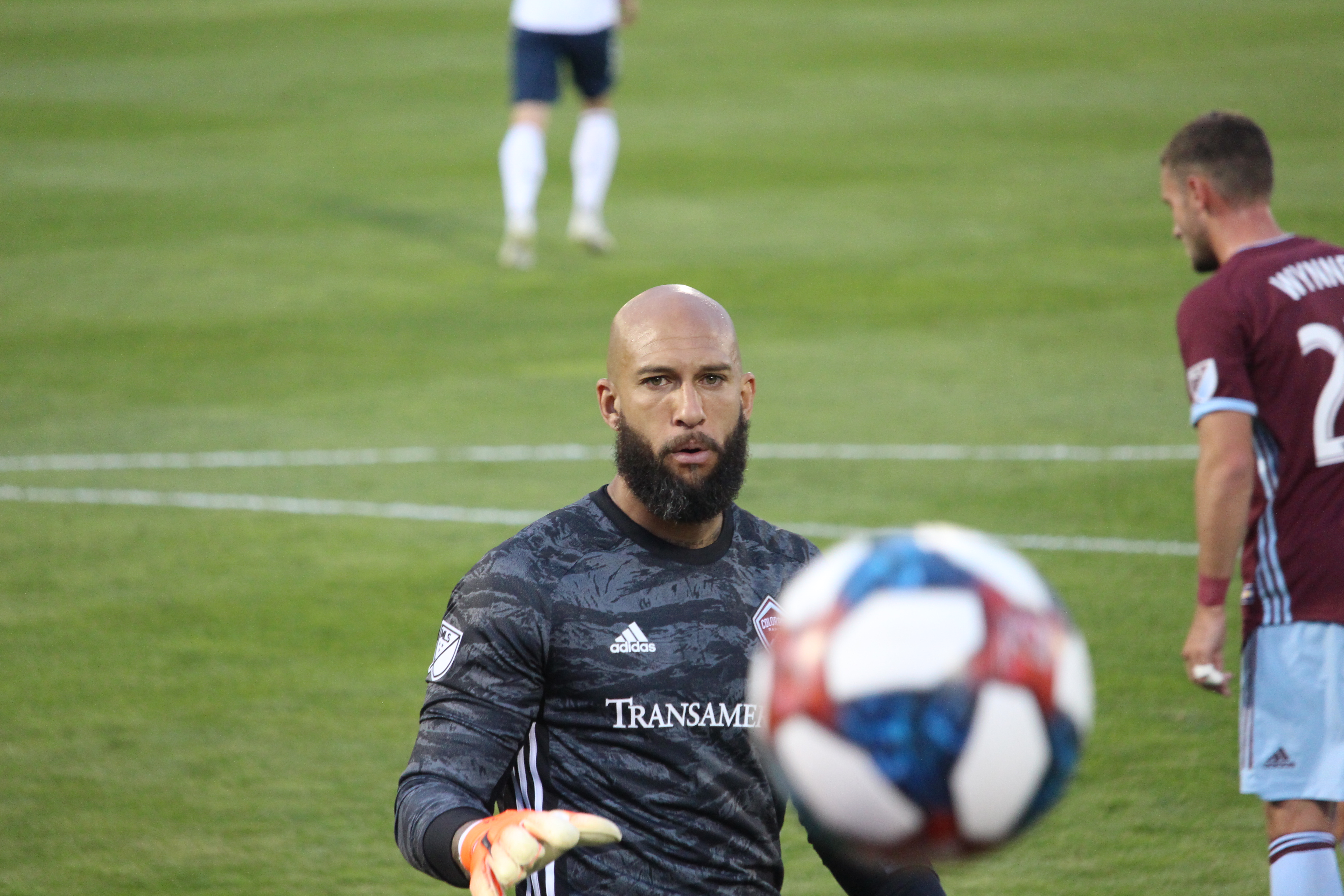This action-packed soccer match photograph features a focused goalie at the foreground center, preparing to catch a vividly colored soccer ball. The goalkeeper, a black man with a brown olive complexion, is bald but sports a thick black beard extending about an inch and a half from his chin. He dons a black and gray camouflage-patterned jersey branded with white Adidas logos, including white stripes under his right arm, and the partially visible "TRANSMERICA" logo across his chest. His outfit is completed with oversized orange and yellow gloves only visible on his right hand. The soccer ball he is eyeing is striking with a white base and complex patterns of turquoise, blue, green, and red shapes that resemble ninja stars or synapses.

To his right, a second player, dressed in a purple jersey with light blue accents, has his back turned to the camera. This white male has a short shaven head and a slight beard, with white tape on his ring and pinky fingers and red tape on his left wrist. His jersey also displays Adidas branding, matching socks, and shorts.

In the blurred background, a third player, likely also white, is seen running away. This person is dressed in solid colors: white socks, blue pants, and a blurry white top, indicating a dynamic game in progress. The green field is marked with white chalk lines, providing context to the sporty scene.